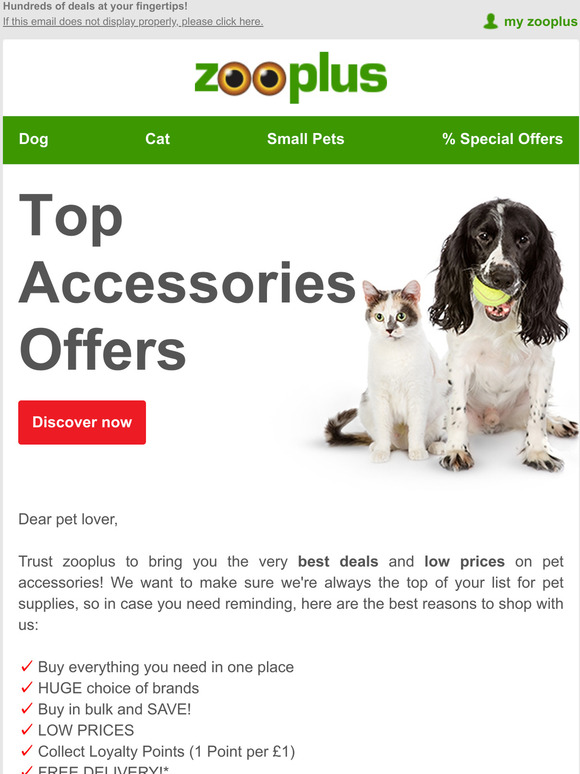In this image, we see a detailed web page for Zooplus, prominently featuring the text "Hundreds of deals at your fingertips." The page appears to be part of a promotional email, as it includes a note stating, "If this email does not display properly, please click here." The headings and categories on the page, such as "My Zooplus," "Dog," "Cat," "Small Pets," "Special Offers," and "Top Accessories Offers," invite the user to explore various sections of the site. There is an encouraging message for pet lovers, explaining why Zooplus should be their go-to choice for pet supplies:

1. Buy everything you need in one place.
2. Huge choice of brands.
3. Buy in bulk and save.
4. Low prices.
5. Collect loyalty points (one point per pound spent).
6. Free delivery.

The color scheme of the webpage uses red, green, brown, black, and white to create an inviting yet professional look. This vibrant palette likely aims to attract pet owners and make navigating the page enjoyable. The image captures the essence of Zooplus's user-centric approach and its commitment to delivering value through a vast selection of pet accessories at competitive prices.